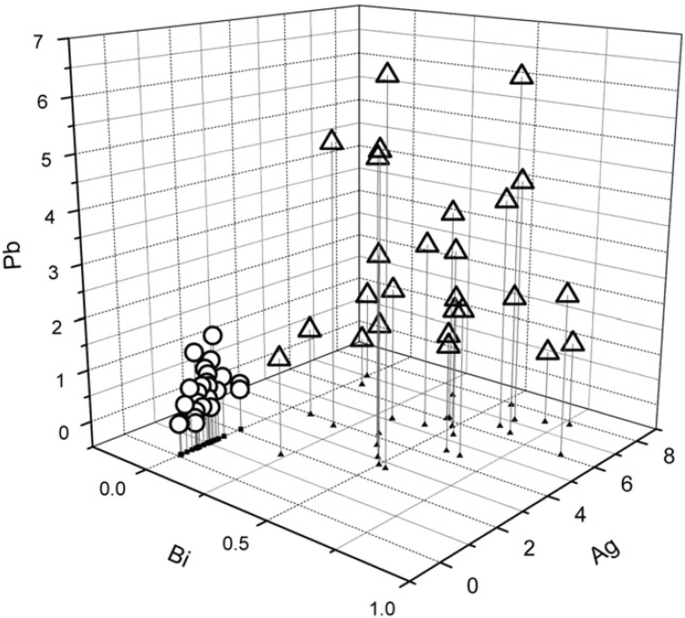The image depicts a black and white three-dimensional graph situated as if within the corner of a room, with visible floor and intersecting walls forming a cube-like frame with the front side removed. The axis to the left is labeled "Pb" and ranges from 0 to 7, the bottom left axis labeled "Bi" ranges from 0 to 1.0, and the bottom right axis labeled "Ag" ranges from 0 to 8. Various lines, both dashed and solid gray, extend from the base grid upwards, connecting to shapes at different levels. Specifically, the lines terminate at either black or hollow triangles and circles. The bottom left features a cluster of gray lines ending in black circle dots, while other sections have these lines topped with circles instead of triangles. The graph's intricate web of lines indicates a complex dataset, visually represented through this detailed three-dimensional structure.